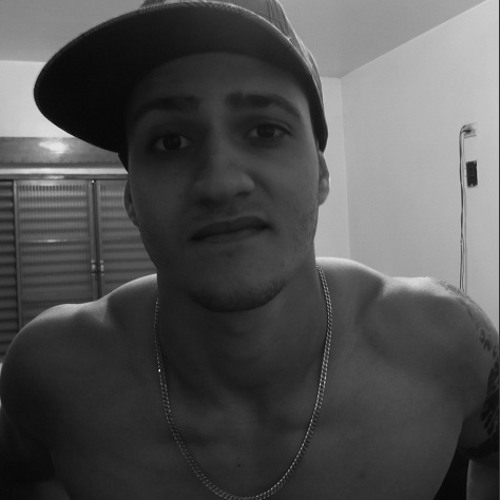The image features a young Hispanic man, likely in his early 20s, standing shirtless in a room with white walls and ceiling. The photo has a grayscale or black-and-white filter. The man is muscular with a tattoo on his left shoulder and arm, and he is wearing a metal necklace. His hat, which appears to cover the top of one of his ears, has a fuzzy or plaid texture. He has a slight goatee and mustache and a neutral expression with a subtly raised right eyebrow and a slight smirk. Behind him to the left, there are closed double doors or a window with shutters, while on the right, there is a plain white wall with some wires visible coming from a high opening. He looks directly at the camera, filling most of the frame from the chest up.